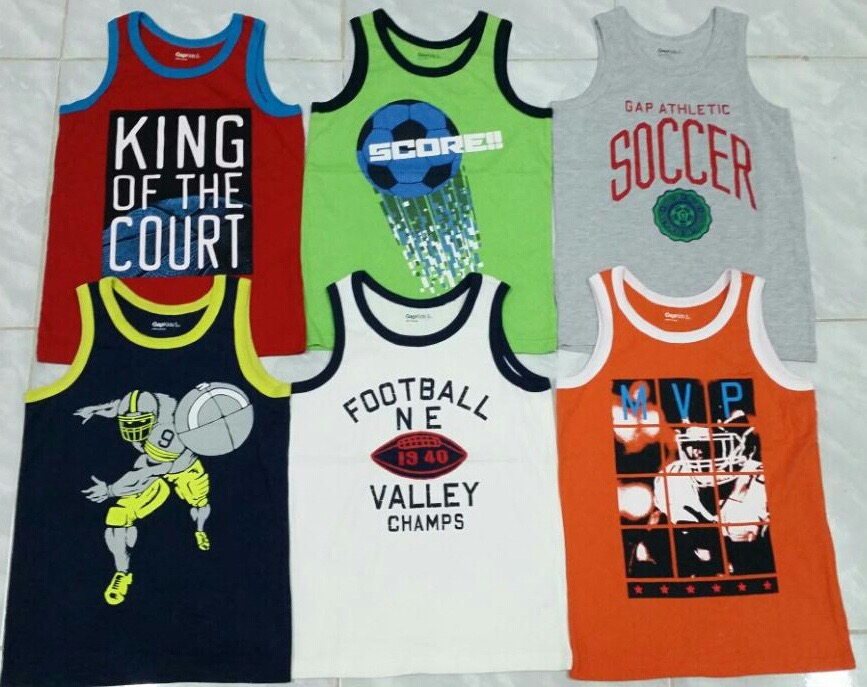This image showcases six sleeveless basketball-style athletic jerseys meticulously laid out on a gray, tiled surface. The arrangement is two rows of three jerseys each. 

1. **Top Left Jersey**: This red jersey features blue trim around the collar and arms. Centered on the jersey, inside a black square, is a basketball image with the phrase "King of the Court" in white text.
2. **Top Middle Jersey**: This jersey stands out with its medium lime green color and black trim. It displays a blue and black soccer ball with silver and gray streaks, giving the illusion of motion. The jersey bears the word "Score!!" in white text.
3. **Top Right Jersey**: A solid gray jersey with red text reads "Gap Athletic" with "Soccer" beneath it. Under the text is a blue and green emblem.
4. **Bottom Left Jersey**: This black jersey has fluorescent yellow trim and features an illustration of a football player in action, detailed with a gray helmet sporting a yellow stripe, a gray shirt with three yellow arm stripes, yellow pants, and yellow shoes.
5. **Bottom Middle Jersey**: This white jersey with black trim displays the text "Football N-E" and has a black and red football graphic with the year "1940" in red print. Below this, "Valley Champs" is printed in black text.
6. **Bottom Right Jersey**: Yellow with white trim, this jersey features a football player and the term "MVP" written in blue. The design is enhanced by a black bar with six red stars.

The consistent elements, such as their sleeveless, scoop-neck design, and placement on a gray tiled background, unify the diverse themes and colors of each jersey.